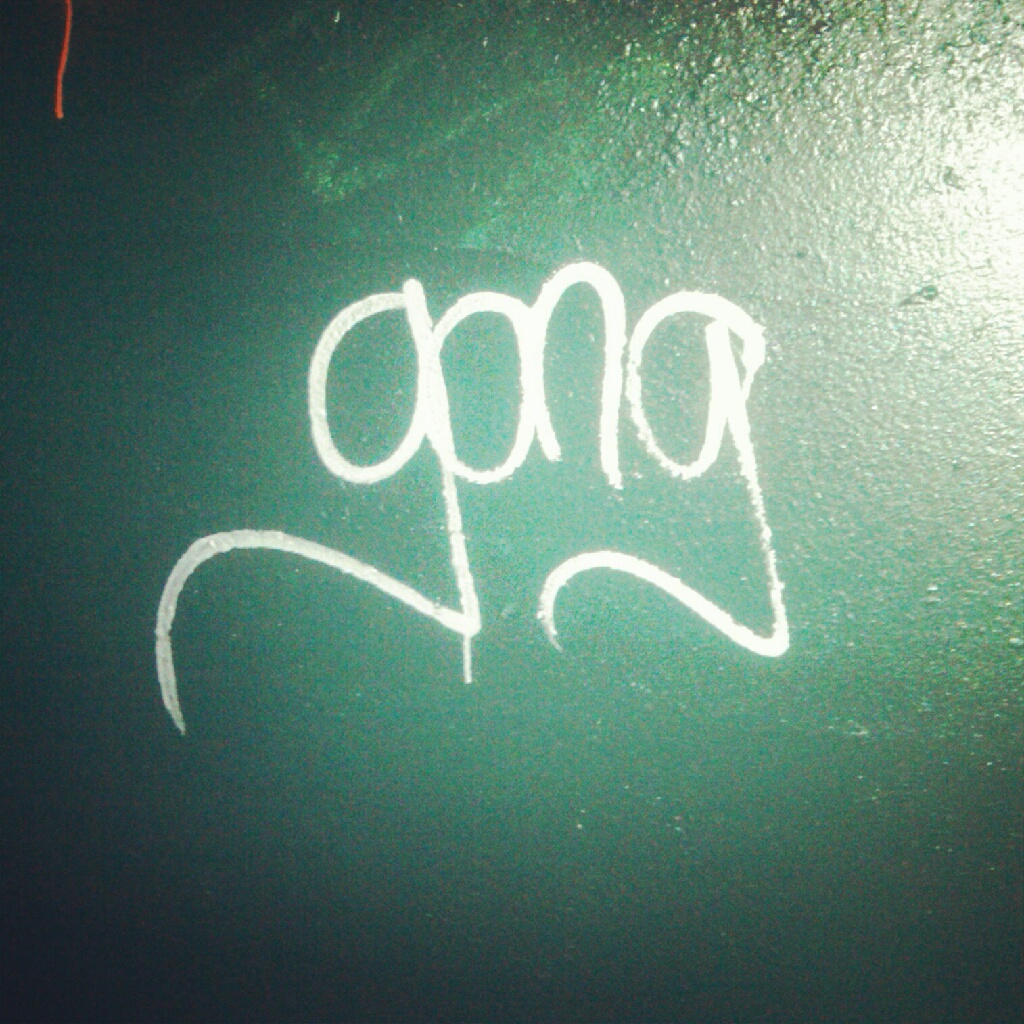This rectangular photograph features a rough, concrete-like wall painted a dark green color. The paint job is inconsistent, revealing some white lines and graffiti near the top that haven't been completely covered. In the top left-hand corner, an orangish-red drip of paint trails down the wall. Dominating the center of the image is a piece of graffiti in white text. There is some ambiguity as the text potentially spells "gang" (G-A-N-G) or "gong" (G-O-N-G), but the former seems more likely. Notable in the text are the lower-case 'g's, which feature curled tails and a dripping effect from the white paint. The photograph also captures some light in the upper right-hand corner, adding a slight glow to that area.